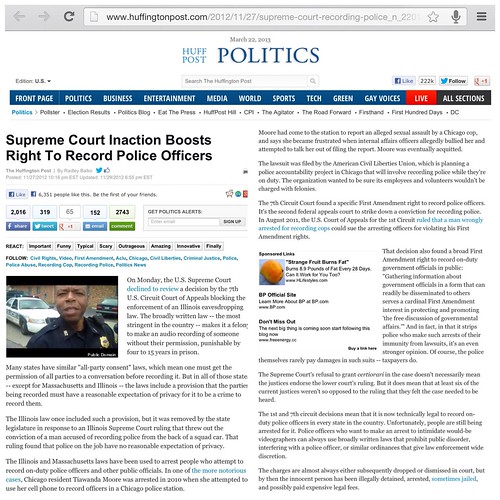This image features a screenshot of the Huffington Post website, as indicated by the URL "www.huffingtonpost.com" displayed in the URL bar at the top of the screenshot. The browser interface displays navigational elements, including a left arrow, right arrow, and a refresh icon on the left side, and a grayish hamburger menu on the right side of the top bar.

Centered prominently on the webpage is "HuffPost" in light blue text, accompanied by the word "Politics" in a dark blue hue to its right. Above these titles, the date "March 22, 2013" is displayed, marking the current date of the content shown.

Directly beneath the main header are several category tabs in white text on a blue background. From left to right, the categories include: Front Page, Politics, Business, Entertainment, Media, World, Sports, Tech, Green, Gay Voices, Live, and All Sections.

The content section below these tabs features articles. The article on the lower left is titled "Supreme Court Inaction Boosts Right to Record Police Officers." Beneath the article title, there are sharing buttons for Facebook, Twitter, and Google, allowing readers to share the story on their social media platforms.